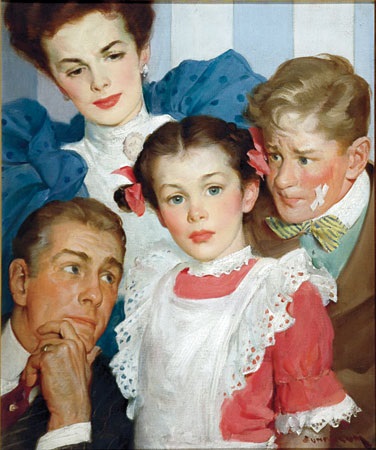This painting depicts a realistic, historical scene set against a backdrop of blue and white striped wallpaper. At the center is a young girl with brown hair styled into side buns, adorned with pink bows. She is wearing a white apron-like dress with pink sleeves and floral designs, complete with lace edges and a white collar. Her dress is highlighted by delicate, lacy ruffles on the short sleeves. Her blue eyes gaze directly at the viewer, giving an impression of innocence.

Behind her, slightly to the left, stands a stern-looking woman with fair skin and reddish hair pulled back into a beehive. She is dressed in a late 19th-century style outfit featuring blue, puffy, ruffled shoulders, white polka dots, a white turtleneck, and a brooch at her neck. She appears to be giving an 'evil eye' to a boy standing next to her.

This boy, an older lad with sandy blonde hair, has a conspicuous white X-shaped tape on his cheek, suggesting he might have been injured. He is wearing a brown suit with a yellow and blue bow tie, a green vest, and a blue shirt, with a slightly reddened cheek adding to his look of consternation.

Seated in the lower left of the painting is an older gentleman, sophisticated and contemplative. He has brown hair, a red tie, a white-collared shirt, and a black suit jacket. He wears a ring on his finger and rests his head on his hand while looking up at the young girl at the center, adding a depth of emotion and curiosity to the scene. Each figure's expression and attire contribute to the intricate storytelling of the artwork.